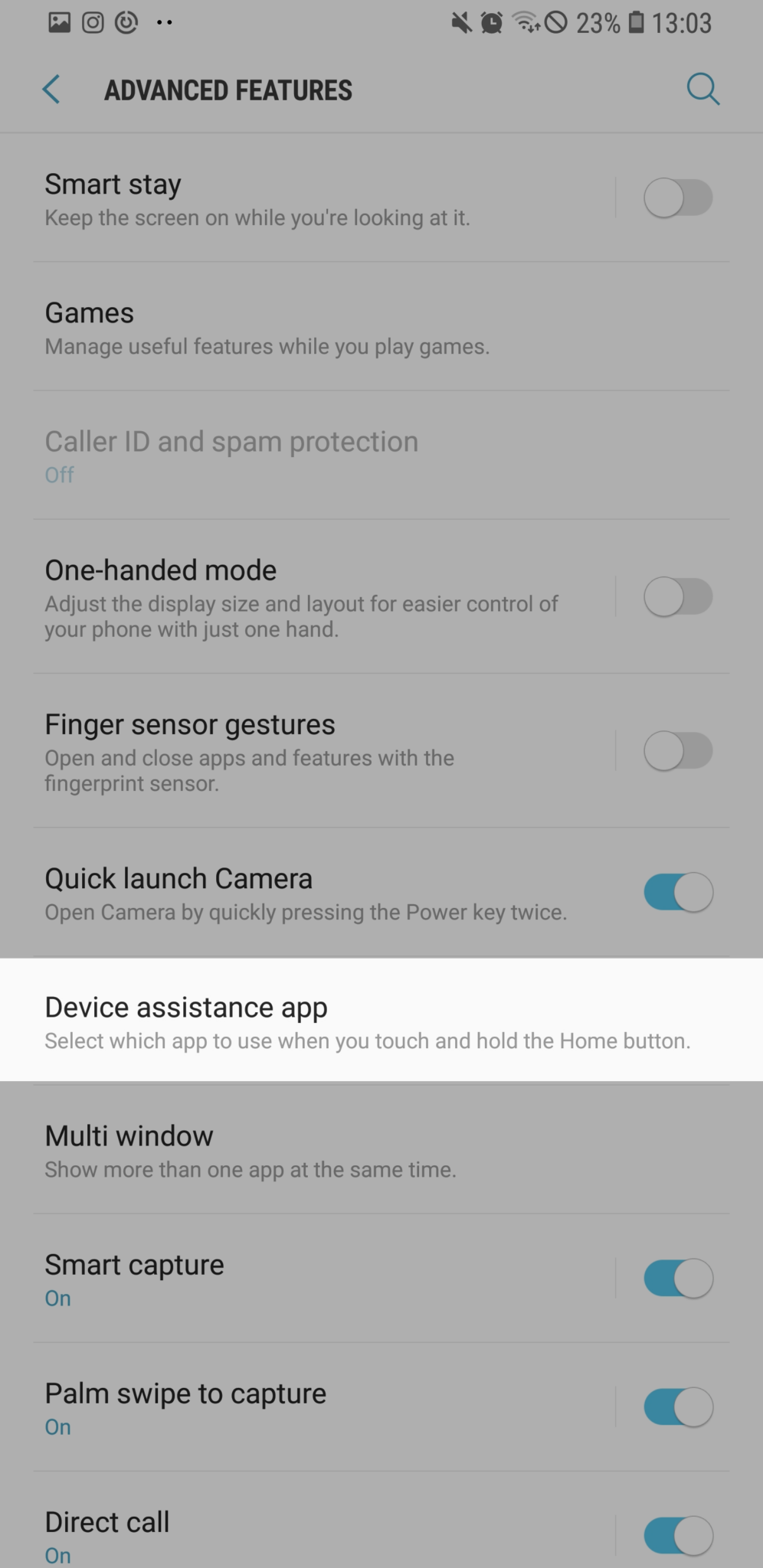This image is a screenshot taken from a cell phone, showcasing the settings menu under "Advanced Features." The background is predominantly gray except for a white section labeled "Device Assistance App," which instructs the user to select an app for the home button assist feature. At the top, a blue search icon is prominently placed next to the "Advanced Features" title.

Below, several options are listed, each accompanied by toggles or status indicators:

- **Smart Stay:** This feature, which keeps the screen on while the user is looking at it, is turned off, as indicated by its gray toggle.
- **Games:** No specific details provided for this option in the screenshot.
- **Caller ID and Spam Protection:** This feature is off, noted by a small blue "Off" label instead of a toggle.
- **One-handed Mode:** This option is turned off, shown by its gray toggle.
- **Finger Sensor Gestures:** This is also turned off, indicated by the gray toggle.
- **Quick Launch Camera:** This feature is enabled, as seen by the blue toggle.
- **Multi-Window:** Listed but not detailed further.
- **Smart Capture:** This feature, along with "Palm Swipe to Capture" and "Direct Call," are all turned on, indicated by blue toggles.

The mixture of gray and white backgrounds aids in distinguishing between different sections and settings within the menu.